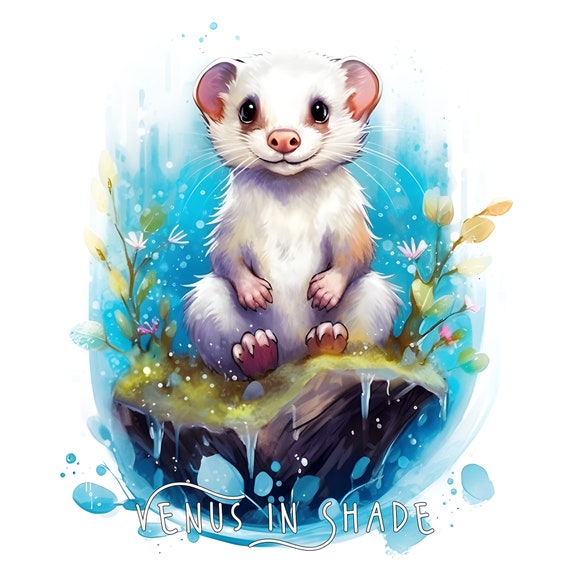This image features a soft painted depiction of a small, white, furry creature that appears to be a baby bear or perhaps a mouse-ferret hybrid. The creature has distinctive black or brown eyes, pink ears, a pink nose, and pink hands and feet. It sits upright on a green patch of grass adorned with budding white and pink flowers, which is situated atop a brown tree trunk. The green patch seems raised, giving the impression of a small cliff. Surrounding the creature are elements of a watery environment, including blue water and water droplets, possibly representing rain. The entire scene is set against a plain white frame with a blue background speckled with white spots. Below the scene, in white text, appears the caption "Venus in Shade," with stylistic features such as an extended 'V' over the word 'Venus' and a curved 'S' in 'Shade.'